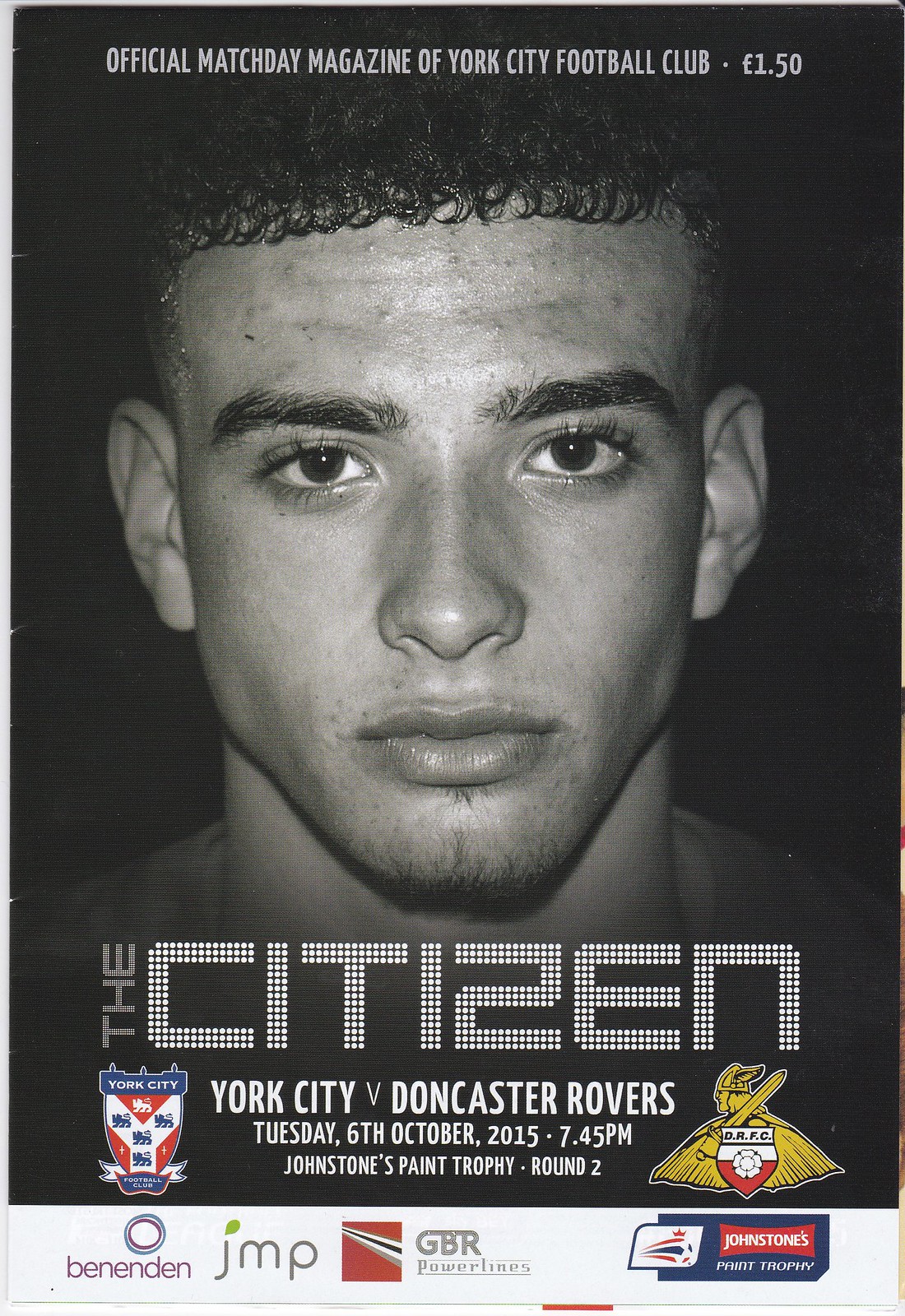This is a cover of an official matchday program for York City Football Club, featured on a black background. At the forefront, there is a striking black-and-white headshot of a young man with short black hair that curls at the front, dark eyebrows and eyelashes, and some chin facial hair. Light reflects off his forehead, adding depth to the image. Above his head, in small white text, it reads, "Official Matchday Magazine of York City Football Club, £1.50." The magazine's title, "The Citizen," is prominently displayed below his chin in a dot font made of small circles. Further text beneath the title provides details of the match: "York City vs Doncaster Rovers, Tuesday 6th October 2015, 7.45pm, Johnstone's Paint Trophy Round 2." 

To the left, there's the York City shield logo, with a Y-shaped design in white set against a red background. On the right-hand side at the bottom, there's a shield logo for Doncaster Rovers Football Club (DRFC), depicting a Viking holding a sword over its shoulder and wearing a cape. An advertisement strip runs across the bottom of the cover, featuring various sponsor logos, including "Ben and Dan," "JMP" with a leaf design, "GBR Power Lines," and "Johnstone's Paint Trophy" with an image of a football. This detailed compilation emphasizes the key graphical and textual elements of the matchday magazine cover.